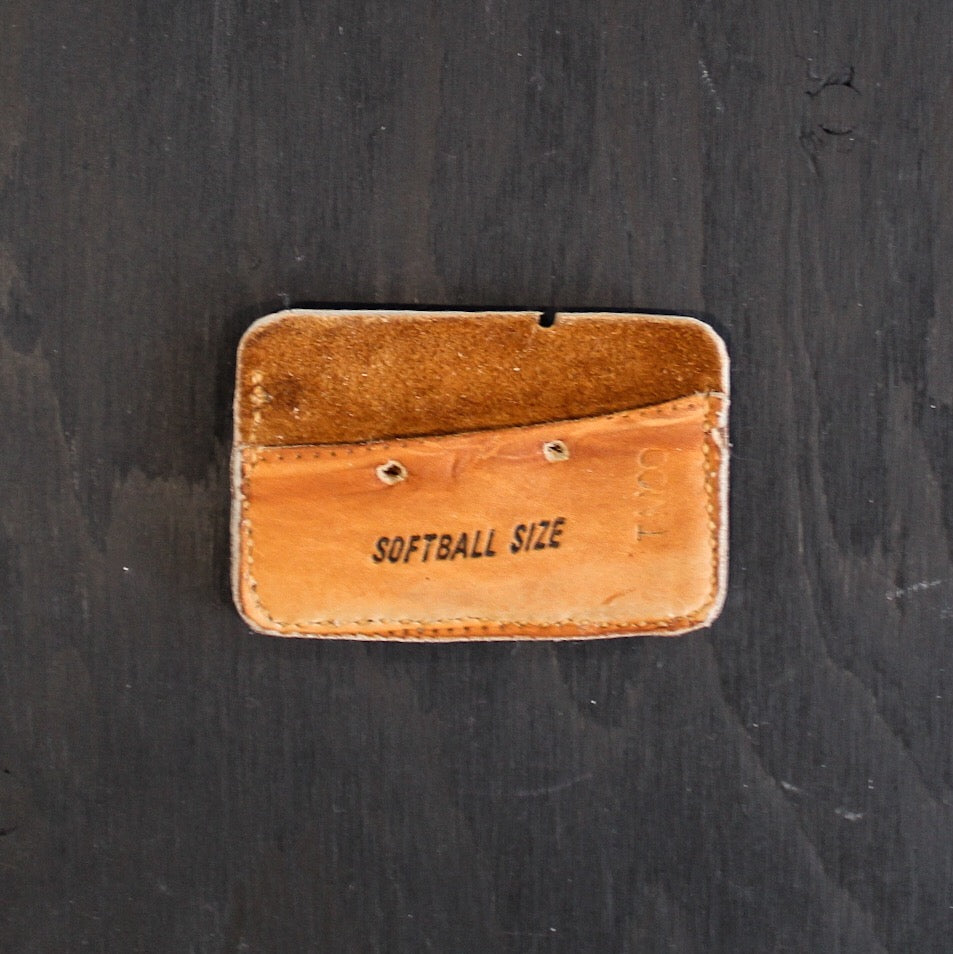In the center of a large square picture, a small, light brown leather pouch resembling a wallet is prominently displayed against a dark wooden surface, which might be a table. The image is taken from above, offering a clear view of the pouch and the textured, wood-like background that appears almost like a tree trunk. The pouch, roughly the size of an old cassette tape, features tan stitching along its sides and bottom. The front side of the pouch is shorter than the back, revealing a suede interior at the top. Two manually punched holes are situated near the top of the front side. The words "SOFTBALL SIZE" are prominently printed in black font on the surface of the pouch. The leather appears slightly worn, adding a vintage feel to the overall composition.